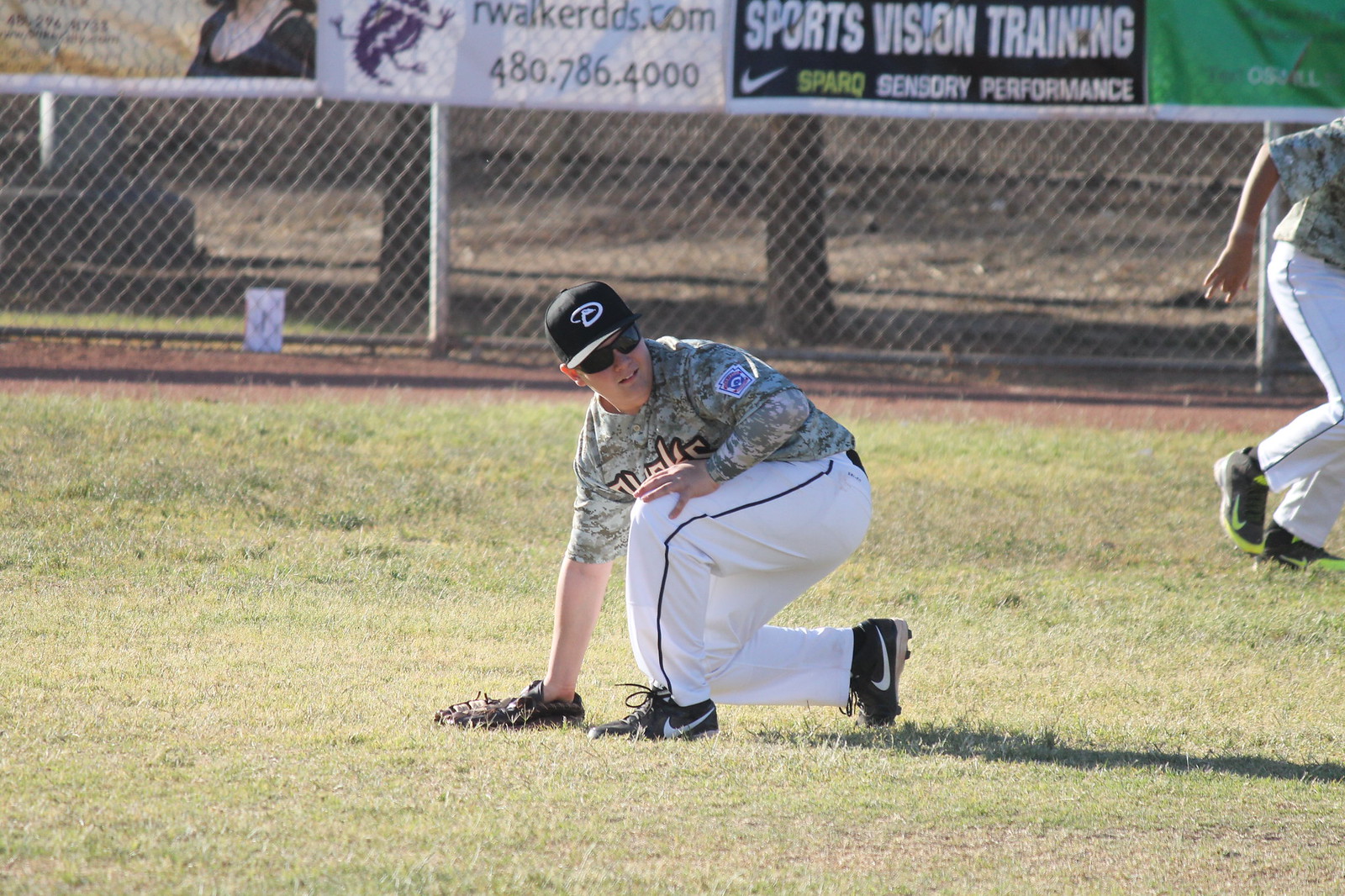The photograph captures a daytime outdoor baseball game, set on a grassy field that appears to be right field. The image is approximately six inches wide and four inches tall. At the center, a player is kneeling on the green grass, facing to the left while looking back towards the right. This individual is dressed in white baseball pants with a black stripe on the side, a green camouflage long-sleeve top with illegible yellow print outlined in black, and Nike cleats. His right hand, which is gloved with a catcher's mitt, rests on the ground. 

Behind him, there's a chain-link fence running horizontally, adorned with one or two banners, including one from "Sports Vision Training." Beyond the fence, a forested area is partially visible. To the far right, the backside of another player, dressed similarly with a baseball cap and glasses, is seen running towards the right. The image has a late-day feel, indicated by the shadows on the ground, adding a sense of time to the lively scene.